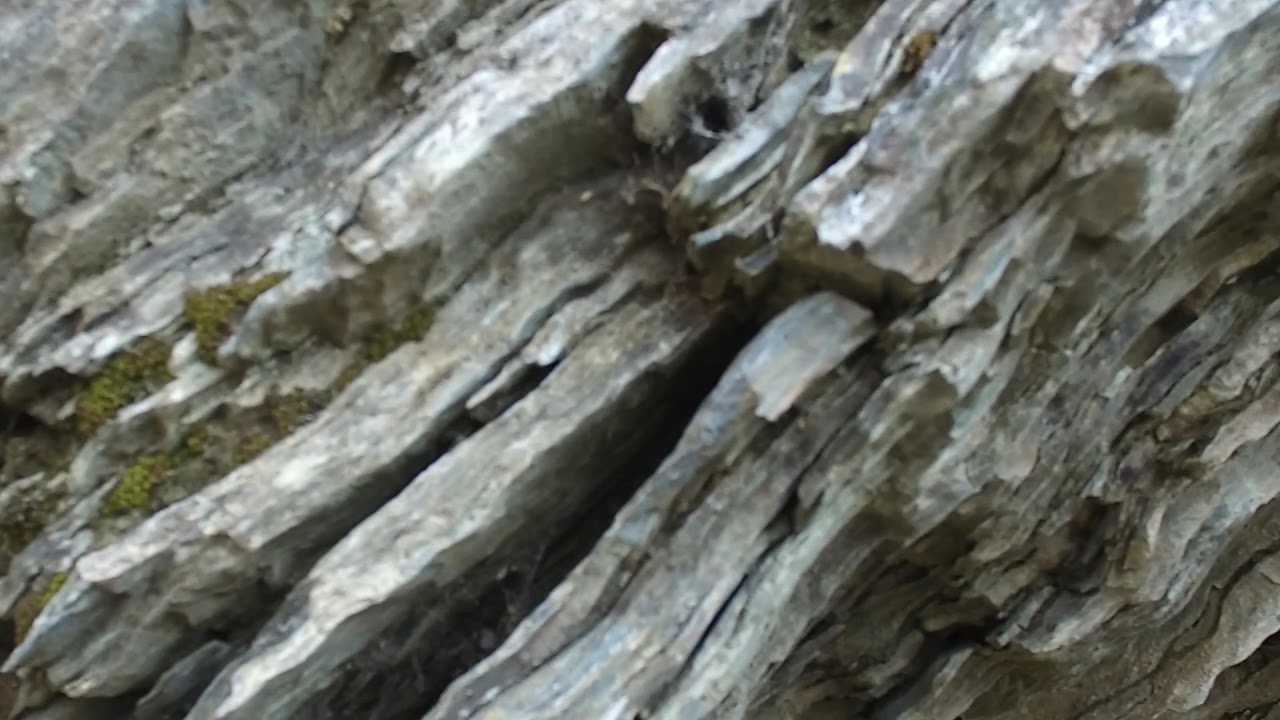The image showcases a close-up of rock formations that resemble the texture and structure of wood or tree bark, akin to petrified wood, situated on what appears to be the side of a mountain range or cliff. The photo, despite its blurry quality, captures intricate details of the rocks which are grayish-brown and exhibit a crumbly, slate-like appearance with long, diagonal patterns. The rocks feature interesting, craggy designs with some regions covered in green moss, especially around the crevices that run diagonally across the image. The presence of moss or possibly shrubs adds a touch of green against the predominantly gray and white rocky backdrop. The entire frame is filled with these textured rock formations, devoid of any people or text, emphasizing the rugged and raw natural beauty of the scene.